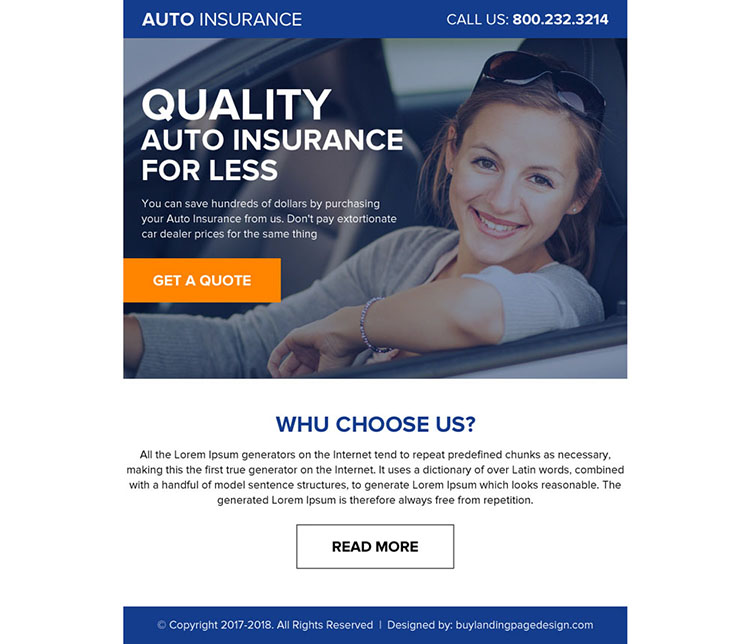The image features a promotional webpage for auto insurance, characterized by a structured and vibrant layout. At the very top of the page, a blue border spans across, bearing the text "Auto Insurance" on the upper left. On the upper right, it says "Call us: 800-232-3214."

Beneath this header is a photograph occupying the main section of the page. To the left of the photo, in large, white text reads, "Quality Auto Insurance for Less." Below this bold statement, in smaller text, it elaborates: "You can save hundreds of dollars by purchasing your auto insurance from us. Don't pay extortionate car dealer prices for the same thing." Adjacent to this description, there's a green and orange rectangle with white text that invites visitors to "Get a Quote."

The background photograph captures a cheerful woman sitting in a car with the driver's window down. She is leaning her elbow on the open windowsill, smiling warmly at the camera. Her longer brown hair is tucked behind her ears, and she has sunglasses perched on top of her head. She accessorizes with a bracelet on her bare left wrist, contributing to her casual, inviting appearance.

Below the photograph is a section titled "Why Choose Us?" The text here is placeholder Latin (lorem ipsum), typically used to simulate actual content. It mentions that all lorem ipsum generators on the internet tend to repeat predefined chunks, yet this particular generator utilizes a dictionary of over Latin words and model sentence structures to create reasonable-looking lorem ipsum text that is free from repetition.

At the very bottom of the section, there is a white rectangle centered with text inviting further engagement: "Read More."